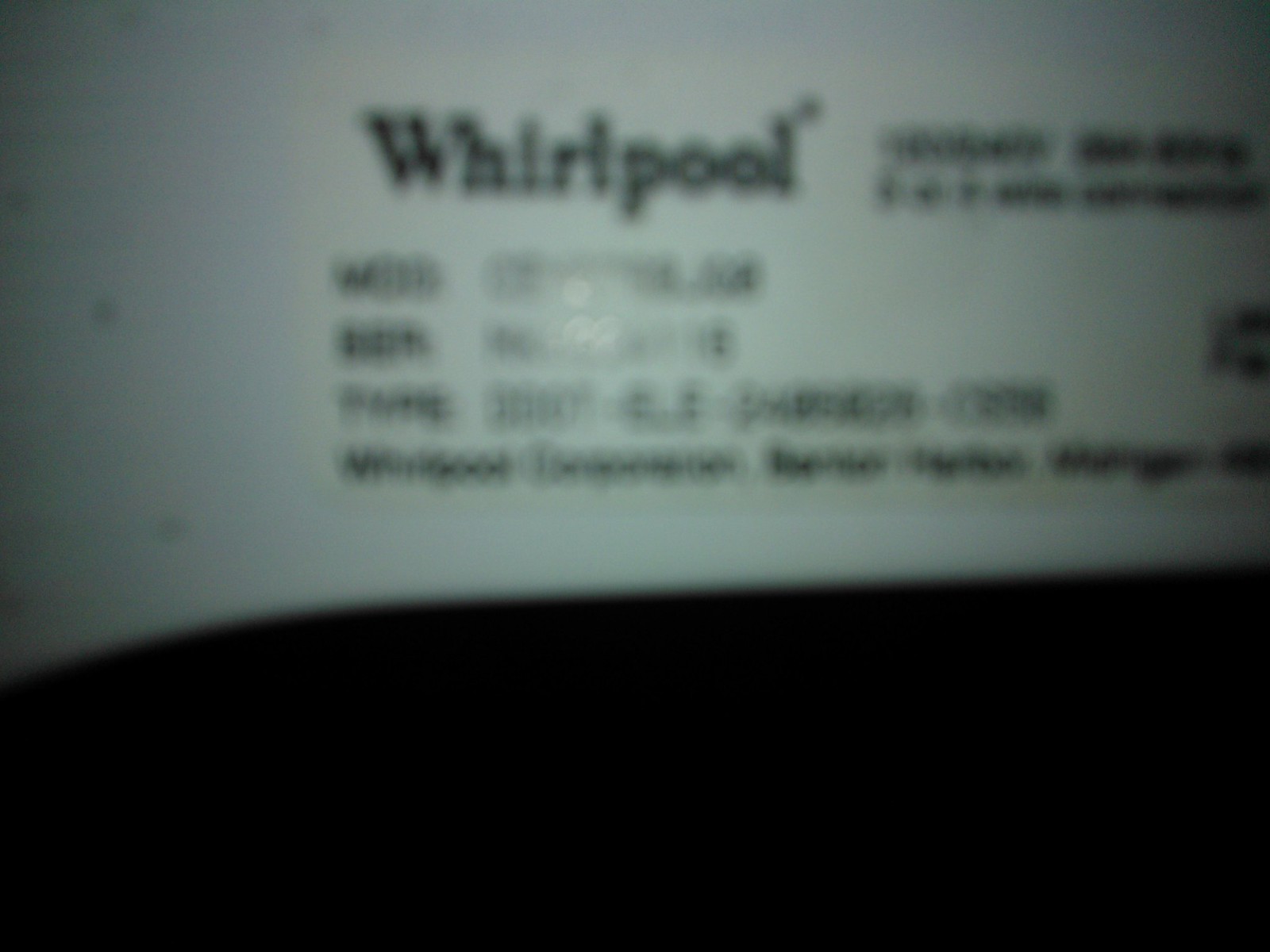This image, taken indoors, is a blurry and low-resolution snapshot of a Whirlpool appliance's product label. The appliance, which could be either a clothes washer or a dishwasher, features a white finish with the Whirlpool brand name prominently displayed in a stylized font. Below the brand name, there is additional text that includes a serial number and other product details, but the blurriness renders this information illegible. The bottom portion of the photo is enveloped in blackness, making it difficult to discern whether it is part of the appliance or merely the background.